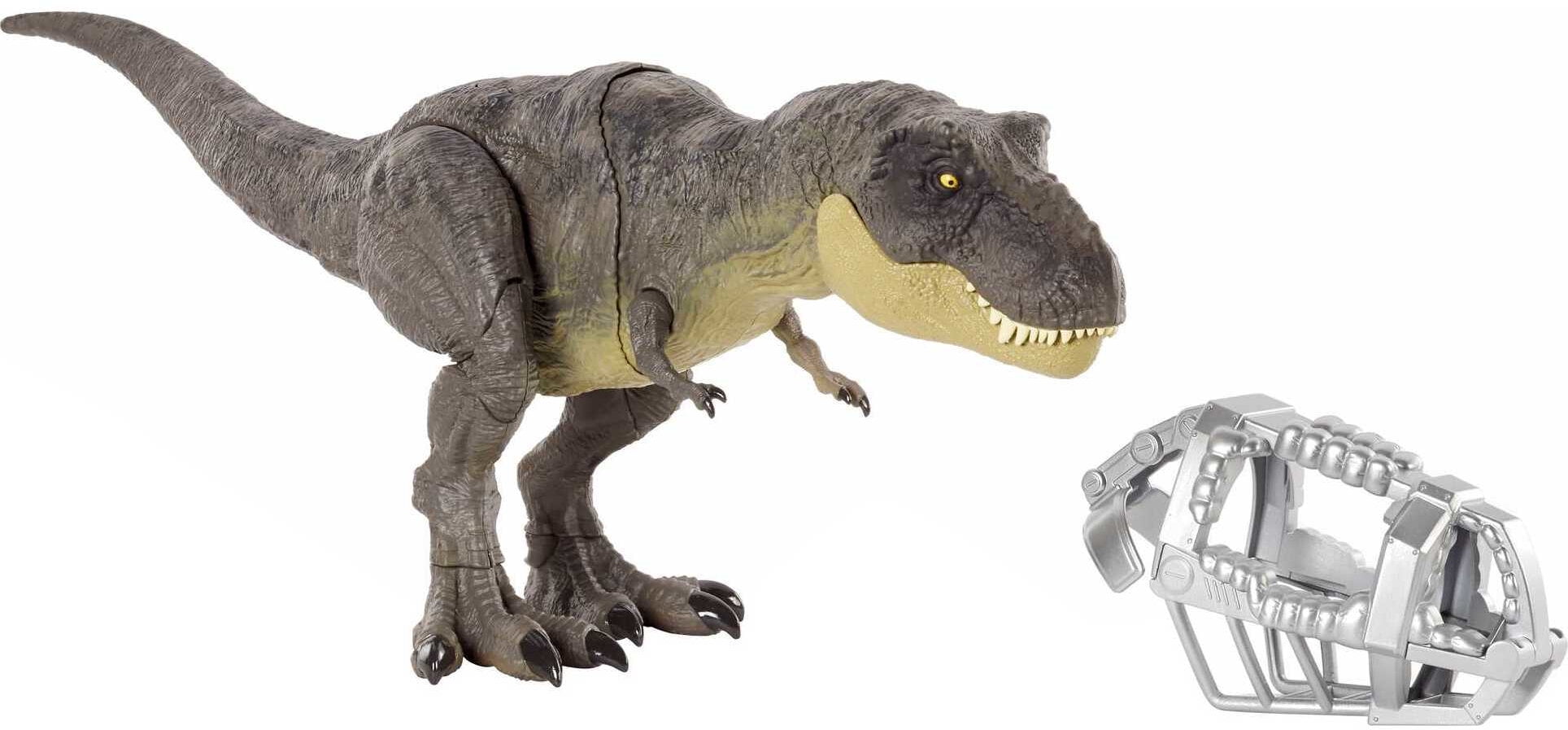The image depicts a highly realistic 3D model of a Tyrannosaurus rex toy, crafted from plastic. The T-rex features a grayish-brown coloration with a tan underside, prominent white teeth, and small yellow beady eyes. It stands upright on its large hind legs with three black-clawed toes, balancing itself with a long tail extending to the left side of the image. Its small arms also possess two black claws each, and its joints are articulated at the knee, foot, and possibly at the jaw. Adjacent to this imposing toy dinosaur is an intricately designed, metallic-looking T-rex muzzle, reminiscent of a pen-and-ink illustration. This muzzle comprises a cage-like structure for the nose and a strap designed to fit around the dinosaur's head, further emphasizing the lifelike and somewhat menacing appearance of the scene.